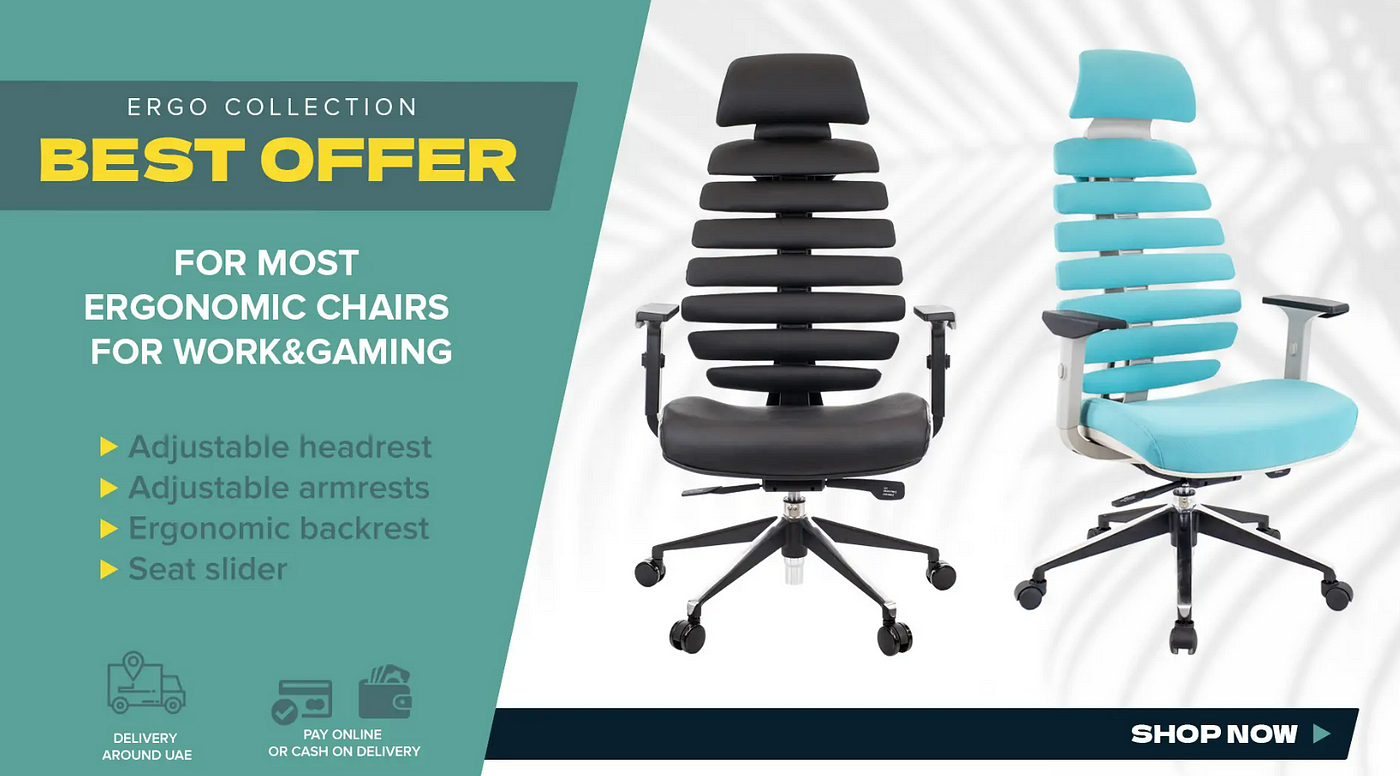The advertisement is a horizontal rectangle divided into two primary sections. The left side features a turquoise trapezoid background, with a darker turquoise trapezoid overlay that prominently showcases the text "Ergo Collection Best Offer" in bright yellow. Beneath this, the text continues to highlight, "For Most Ergonomic Chairs for Working and Gaming," followed by four yellow arrow bullet points listing key features: Adjustable Headrest, Adjustable Armrests, Ergonomic Backrest, and Seat Slider. At the bottom left, logos indicate "Delivery Around UAE" with an image of a truck, accompanied by "Pay Online or Cash on Delivery" with icons of a credit card and a wallet. The right side features a white background with subtle palm frond shadows and showcases two ergonomic chairs. The left chair is black with matching cushions, backrests, and headrests, while the right chair has light blue cushions, backrests, and headrests. Both chairs include armrests and rolling wheels. In the bottom right corner, a black rectangle with white text reads "Shop Now."